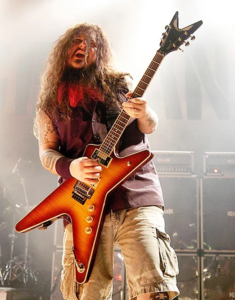This is a full-color, close-up photograph taken indoors under artificial lighting at a rock concert. The vertically rectangular image captures the late Dimebag Darrell, the renowned guitarist from Pantera. His long, wavy brown hair cascades over his face, partially obscuring it. Dimebag is attired in a sleeveless black or dark-colored tank top and khaki cargo shorts that stop just above his knees. His arms are adorned with tattoos, and he sports a maroon sweatband on his right wrist. Notably, he has a soul patch beard and is a white man.

Dimebag is engrossed in playing his distinctive Gibson Flying V guitar, which features a light-colored orange center with darker orange and reddish tones along the edges. The guitar's body has an X-like shape with a truncated top-left leg and a V-shaped top. The background is blurred and smoke-filled, with large black speakers and transport trunks visible, indicating the concert setting. A wash of bright light from above illuminates the scene, adding to the vibrant, electric atmosphere of the performance.